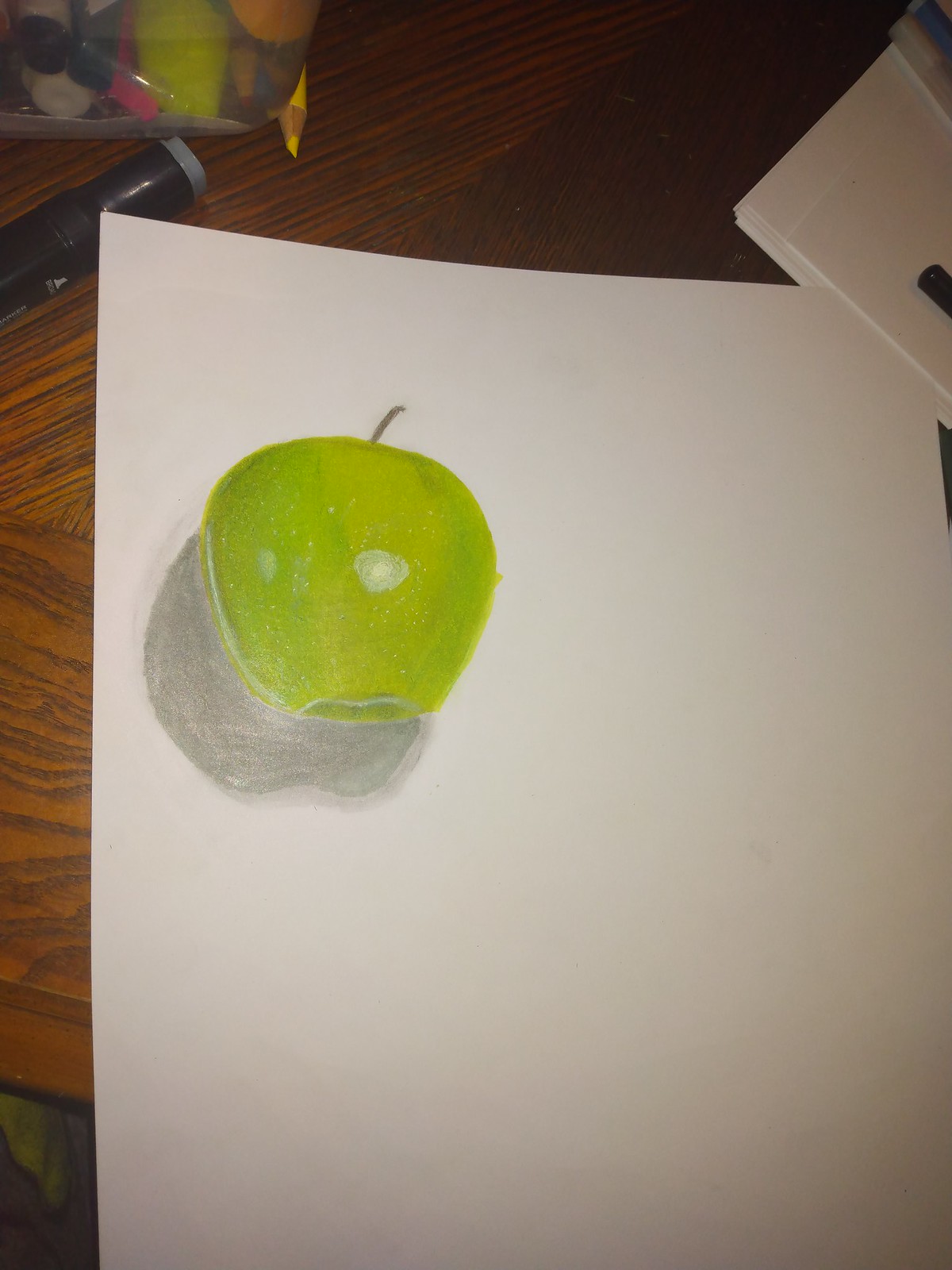A detailed and intricate artist's sketch of a medium green apple is prominently showcased in the upper left corner of an off-white sheet of art paper. The apple is meticulously rendered, complete with speckles, imperfections, and a dark green stem, giving it a realistic appearance. There is a distinct shiny spot in the center of the apple, highlighting its texture. Behind the apple, a grayish-green shadow is artfully added, likely using a pencil or crayon, enhancing the depth of the sketch.

The entire composition rests on a rich walnut wood grain surface. In the upper right corner of the image, additional sheets of paper are visible, along with the top of a drawing pencil or pen. In the upper left corner, another pen lies on the surface, suggesting an ongoing creative process. The use of colored pencils or crayons imbues the apple with a soft, blended edge, showcasing the artist's skill in bringing the fruit to life.